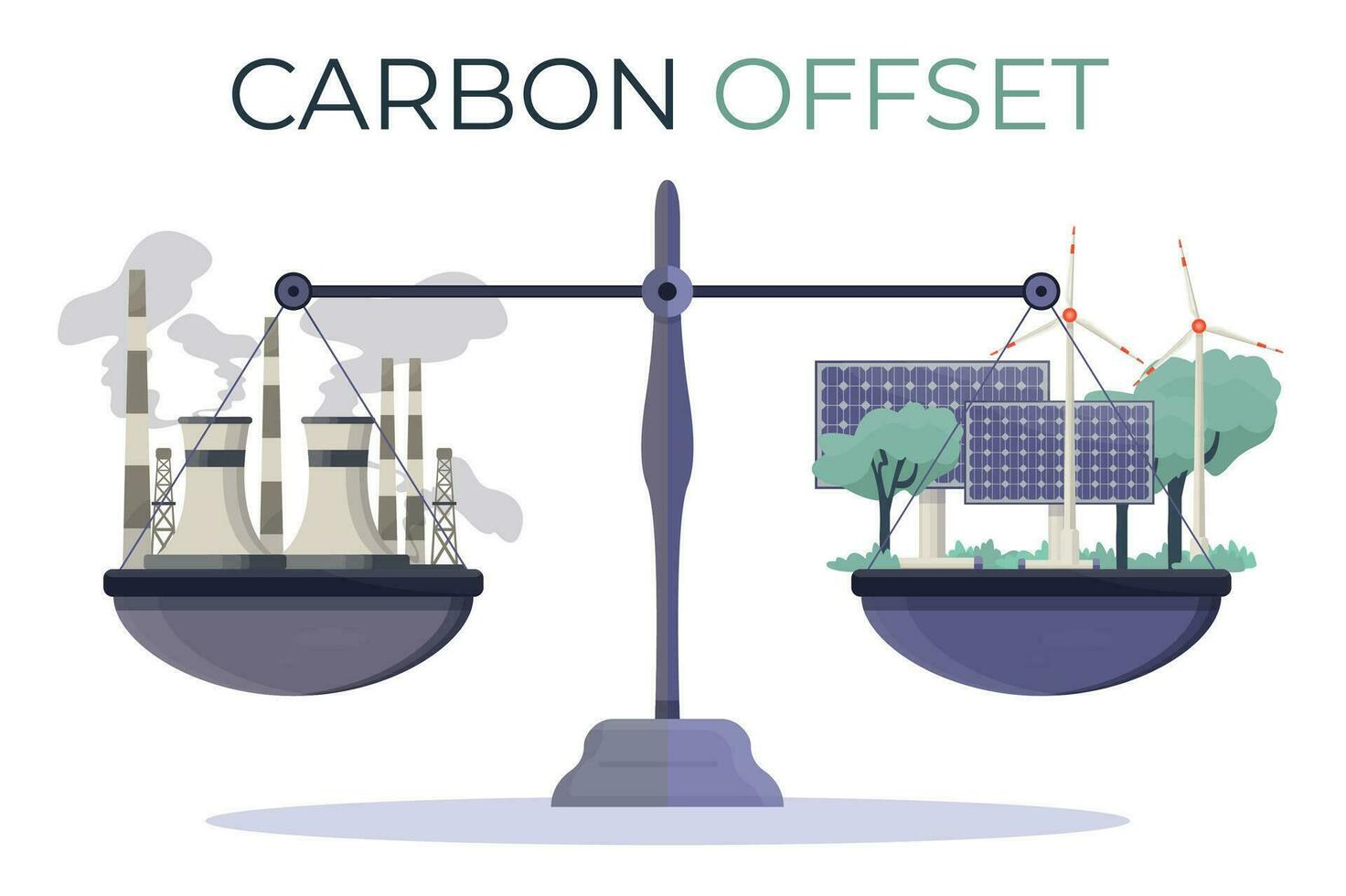The image features a prominent weighing scale set against a stark white background, with a subtle elongated oval shadow beneath it. The scale is gray, consisting of a central stand with two pans extending outward. At the top of the image, written in capital letters, are the words "CARBON OFFSET," with "CARBON" in dark blue and "OFFSET" in light blue.

On the left pan, there are several industrial elements, including nuclear cooling towers emitting smoke or steam, oil rigs, and smokestacks. This side is labeled "CARBON," highlighting the negative environmental impact of these energy sources.

On the right pan, the contents are more environmentally friendly. This side holds trees, solar panels, windmills, and grass, representing sustainable energy sources. It is labeled "OFFSET," indicating these elements are intended to counterbalance the carbon output depicted on the left side. 

The detailed and contrasting contents in each pan emphasize the balance and trade-off between carbon emissions and green offsets.